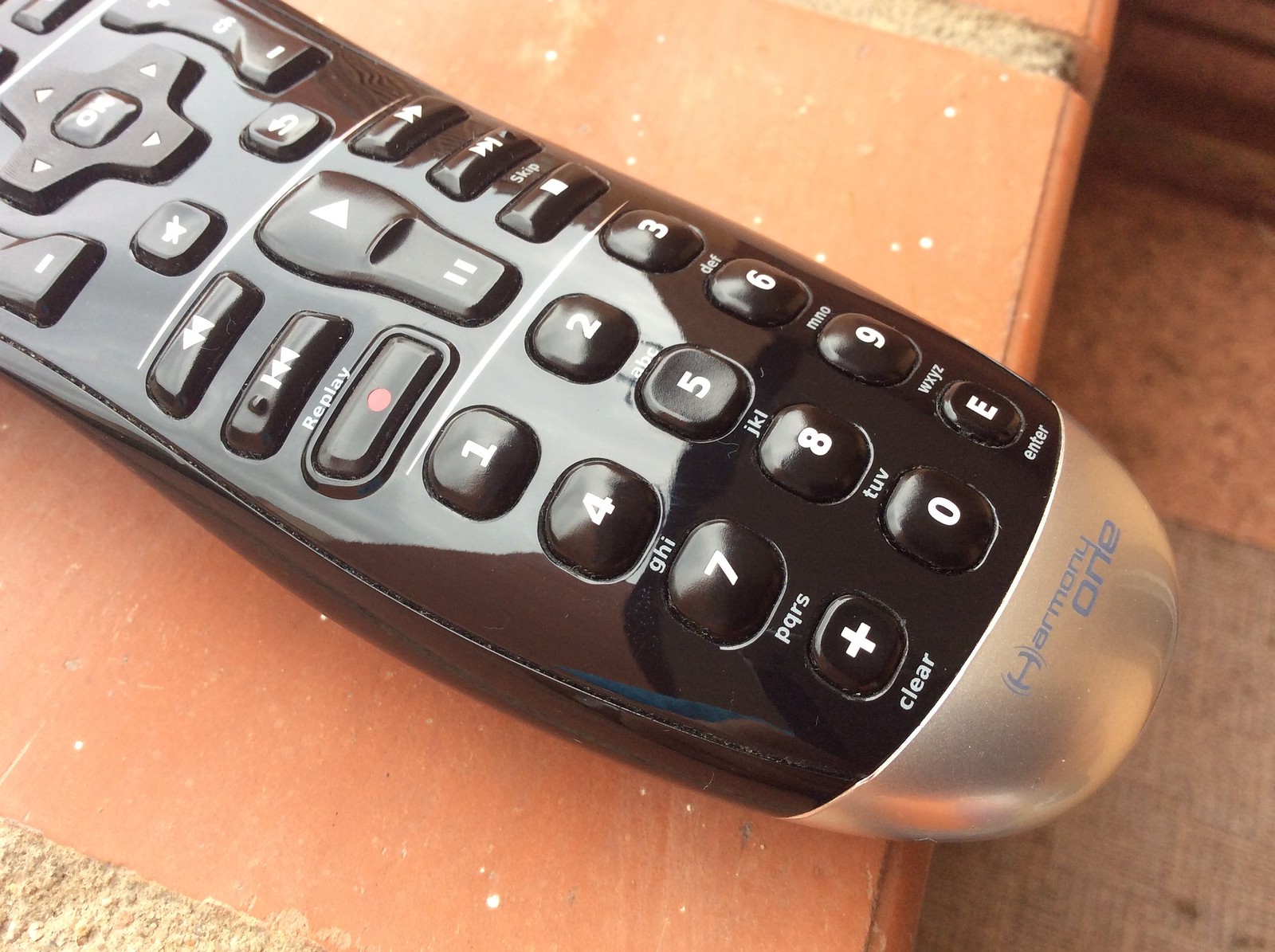The image depicts a close-up of a Harmony One universal remote, resting on a light brown, terracotta-like counter with white grout. The remote's casing is predominantly black or very dark brown plastic, with a matte silver chrome cap at the bottom bearing the pale blue inscription "Harmony One." The visible portion of the remote includes number keys from 1 to 9, each paired with corresponding alphabetical sequences (e.g., ABC under 2, DEF under 3). Under the 9 key, there is a capital "E" labeled "Enter," flanked by a "0" key and a "+" key with the label "Clear." 

Prominently featured in the middle section, there is a circular navigation pad with directional arrows (up, down, left, right) surrounding an "OK" button. Surrounding this pad are various control buttons: a red "Replay" button, rewind, fast-forward, play, pause, and skip buttons, identifiable by their distinct icons. The scene captures an older wooden table with paint splatter in the foreground and a background showing a tiled floor with a gray and pink rug. Only about two-thirds of the remote is visible in the photo, emphasizing its essential controls and distinctive design.